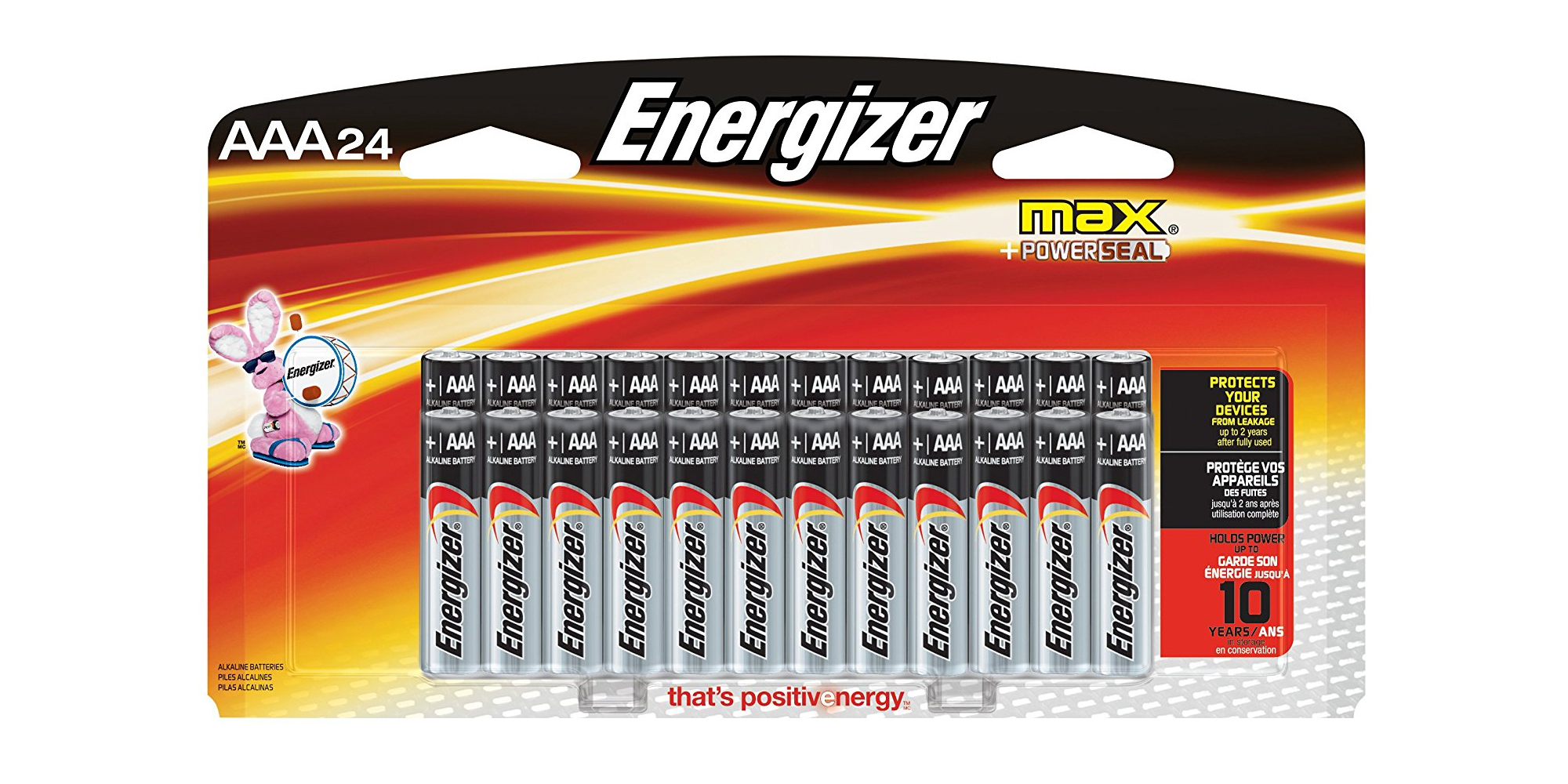This image displays a packet of Energizer batteries, specifically featuring AAA Alkaline batteries. In the bottom left corner, the packet prominently shows the labels "Alkaline Batteries" along with "Alkalines" and "Alcalinas" in multiple languages. The bottom right center of the packaging carries the phrase "That's Positive Energy," with the 'E' from "Positive" rendered in white, seamlessly initiating the word "Energy."

The central section of the packaging displays a neatly arranged grid of 24 AAA Alkaline Energizer batteries. The grid consists of two rows, each containing 12 batteries; the top row shows the entire length of the batteries while only the tops of the batteries in the bottom row are visible. 

Adjacent to the batteries, on the left, is the iconic Energizer Bunny. To the right, there is text indicating the batteries "Protect Your Devices from Leakage for Up to Two Years," along with its French translation. Below this, a black bold text states the batteries "Hold Power for Up to Ten Years."

At the top center, the word "Energizer" is written in white font. The top left corner reads "AAA 24," specifying the battery size and quantity. On the top right, the packet advertises "MAX PLUS Power Seal." The background image of the packaging features traditional Energizer colors with a vibrant burst of bright orange, yellow, and gold hues, crisscrossing dramatically, almost resembling an explosion concentrated around the "MAX POWER SEAL" text.